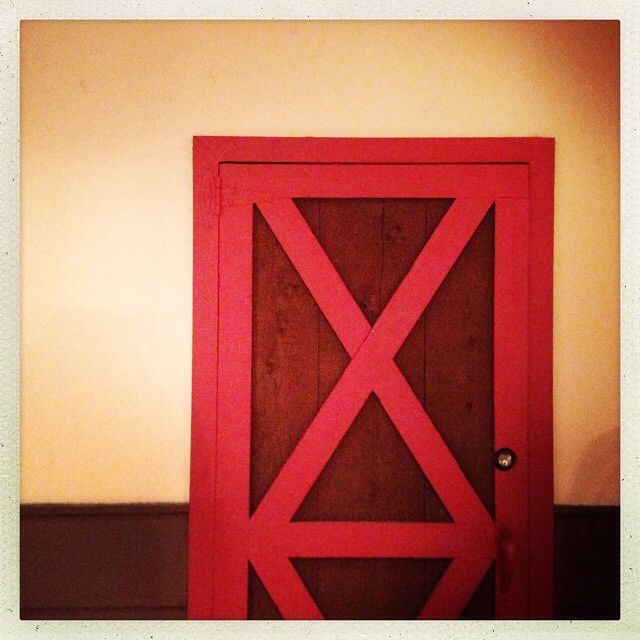The image showcases a detailed close-up of a barn-style door prominently positioned slightly to the right of the center. The door itself features red trim, including a distinct X pattern formed by red planks overlaying four vertically aligned, dark varnished wood slats. A metal handle is visible, hinting at the door's functionality, and there appears to be a circular area that could accommodate a lock, though this detail is somewhat obscured. 

The door is framed by a light gray or tan border, set against a wall that has a chair rail dividing it into two sections: the bottom half in brown and the top half in a very light orange. The scene is further enriched by subtle shadows cast on the wall to the right of the door, adding depth to the composition. The exact setting—whether interior or exterior—is indeterminate, but the barn-like aesthetic suggests a rustic farmhouse environment. The entirety of the image is encased within a white outer border, emphasizing the rustic charm of the focal door.